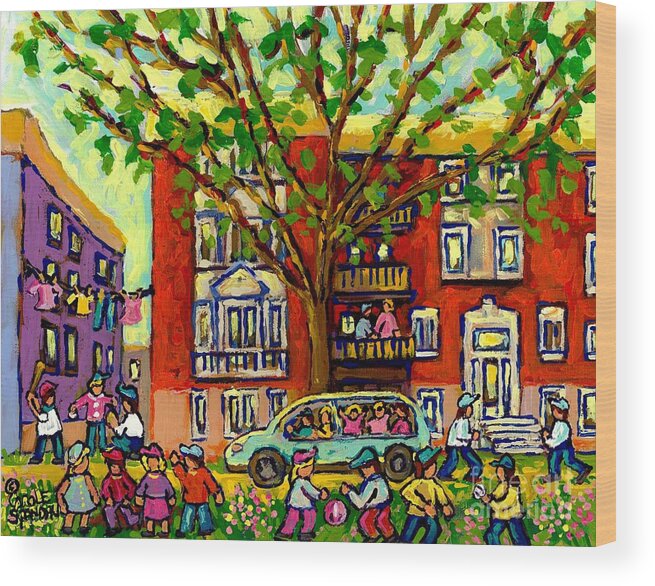This painting illustrates a vibrant neighborhood scene rendered with a childlike artistic style. At the forefront, a group of children, dressed in varied outfits of blue, red, and yellow, are seen playing on a patch of green grass adorned with blossoming flowers. Each child wears a hat, adding to their playful appearance. Central to the composition is a light blue van with large open windows, out of which more children in similar attire excitedly reach and shout. To the left stands a striking purple house with a flat, yellow-topped roof, connected via a clothesline adorned with colorful garments to a broader, red apartment building with yellow window fixtures and multiple patios. On one of these patios, people engage in conversation. To the right of the van, two similarly dressed men walk by. A notable feature of the scene is a large, leafy tree dominating the middle ground, its presence unifying the bustling activity below. Beneath the clothesline stretch two children engaged in a spirited game of baseball, one pitching and the other batting, with a potential umpire standing nearby. Amidst the lively tableau is a signature in black situated towards the left, anchoring this cheerful and detailed snapshot of neighborhood life.